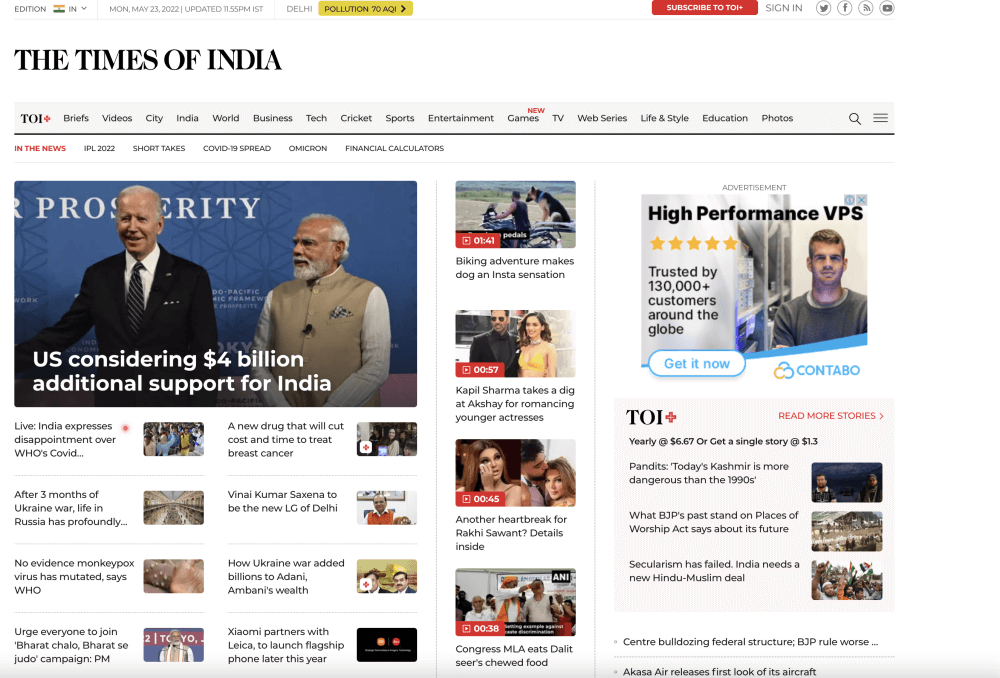This image is a detailed screenshot of the Times of India's online newspaper webpage. At the very top left, the webpage displays "Edition" followed by "Monday, May 23rd, 2022." Next to this, it is indicated that the content was updated at 1:56 p.m. Adjacent to the date and time, it shows the Delhi Pollution level at 70 AQI. To the right of this information, there is a prominent red button labeled "Subscribe," followed by icons for "Sign In," "Twitter," "Facebook," and two other social media platforms.

Beneath the header, the "Times of India" logo is prominently displayed on the left side. Below the logo is a light gray navigation bar including links labeled: TOI, Briefs, Videos, City, India, World, Business, Tech, Cricket, Sports, Entertainment, Games, TV, Web Services, Life & Style, Education, Photos, a search bar, and a menu icon represented by three lines.

The main content section features an image on the left side showing President Biden with the President of India, accompanied by a headline that reads, "U.S. considering $4 billion additional support for India." On the right side of this main content area, there is an advertisement for high-performance VPS, emphasizing its trust by over 130,000 customers globally. Below this, there is a list of various clickable article headlines that readers can explore for more information.